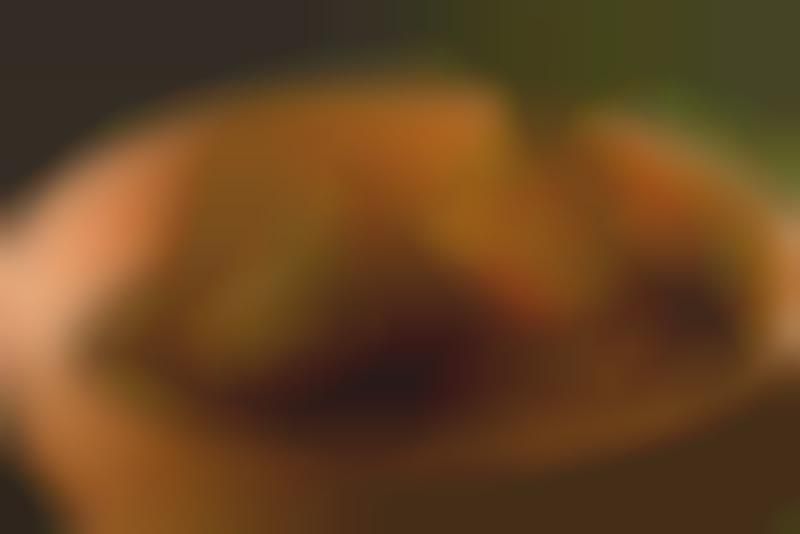A highly blurred and indistinct photograph featuring an elliptical shape at the center, reminiscent of an artist's palette due to a small notch on its top right side, possibly where a thumb would hold it. The elliptical area showcases muted shades of light brown with a hint of red, while its center is a mix of blurry green, dark, and red tones. The overall image's color palette is softened and unclear. The top left corner of the photograph is enveloped in black, transitioning to a green hue towards the top right, creating a gradient effect. The bottom right corner is dominated by dark brown shades, while the bottom left corner presents an even deeper brown in a smaller region.